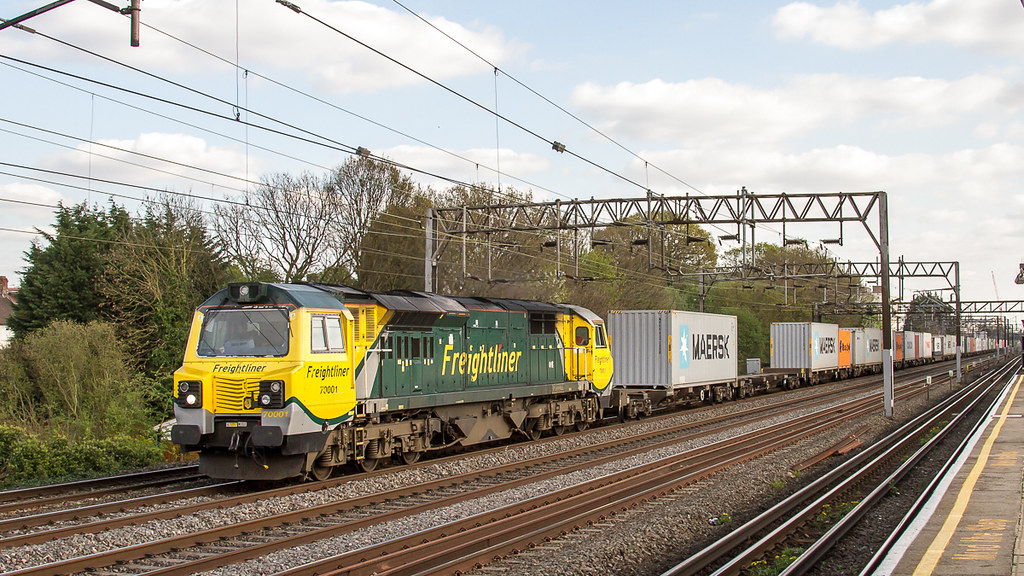The photograph depicts a scene from a train platform, showcasing four sets of train tracks that extend from the bottom left to the top right of the image. The track furthest from the viewer hosts a long, colorful train extending into the distance. This train is distinguished by its yellow and green locomotive, with "Freightliner" emblazoned in yellow text on the green center, and repeated in green text on the yellow front and side sections where the conductor’s cabin is located. The side also displays a series of numbers, likely "7000 0001". Further along the train, various grey containers marked with the MAERSK logo are visible, indicating the train's cargo. Overhead, a network of power and guard lines crisscrosses above the tracks. The backdrop includes green and brown vegetation—plants and trees—that contrasts with the industrial scene. The sky above is bright, dotted with puffy clouds, adding a touch of natural beauty to the otherwise mechanical landscape.